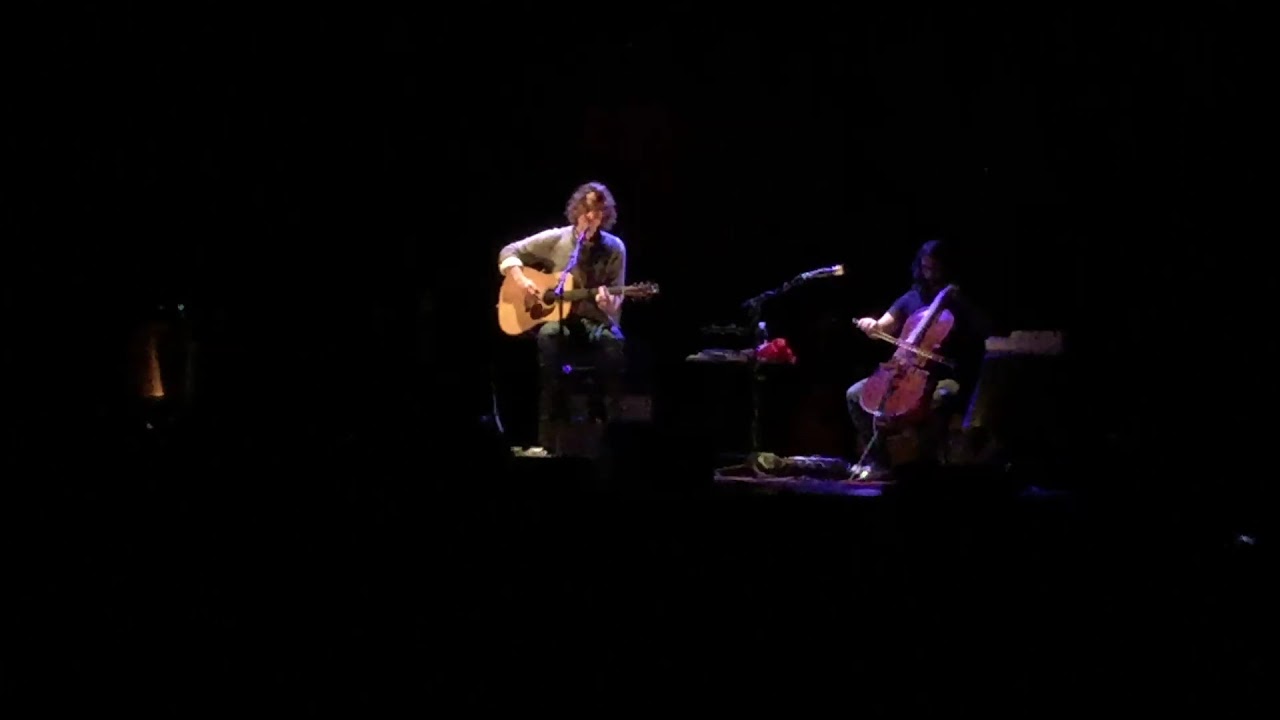The horizontally aligned rectangular picture captures a dark, mostly black backdrop with a subtle streak of light in one corner. At the very center, illuminated by overhead spotlights, stand two musicians. The man in the spotlight to the left is playing an acoustic guitar, with shoulder-length wavy or curly hair, dressed in a grey long-sleeve shirt with rolled-back sleeves and dark pants. His right hand strums the brown, sandal-colored guitar while his left hand grips the strings at the frets. A microphone stands before him, suggesting he might be singing as well. 

To the right of him, slightly further back, another man is playing a violin. He has short hair and wears a dark or blue short-sleeve t-shirt with dark pants. A second microphone is positioned facing another direction. A table with a red object on it sits between them, and the floor features some visible chords. The musicians are framed against a black curtain backdrop, making the scene likely to be either a stage performance or a practice session. The detailed shadows and lighting enhance the musicians' form, focusing all attention on their instruments and performance.